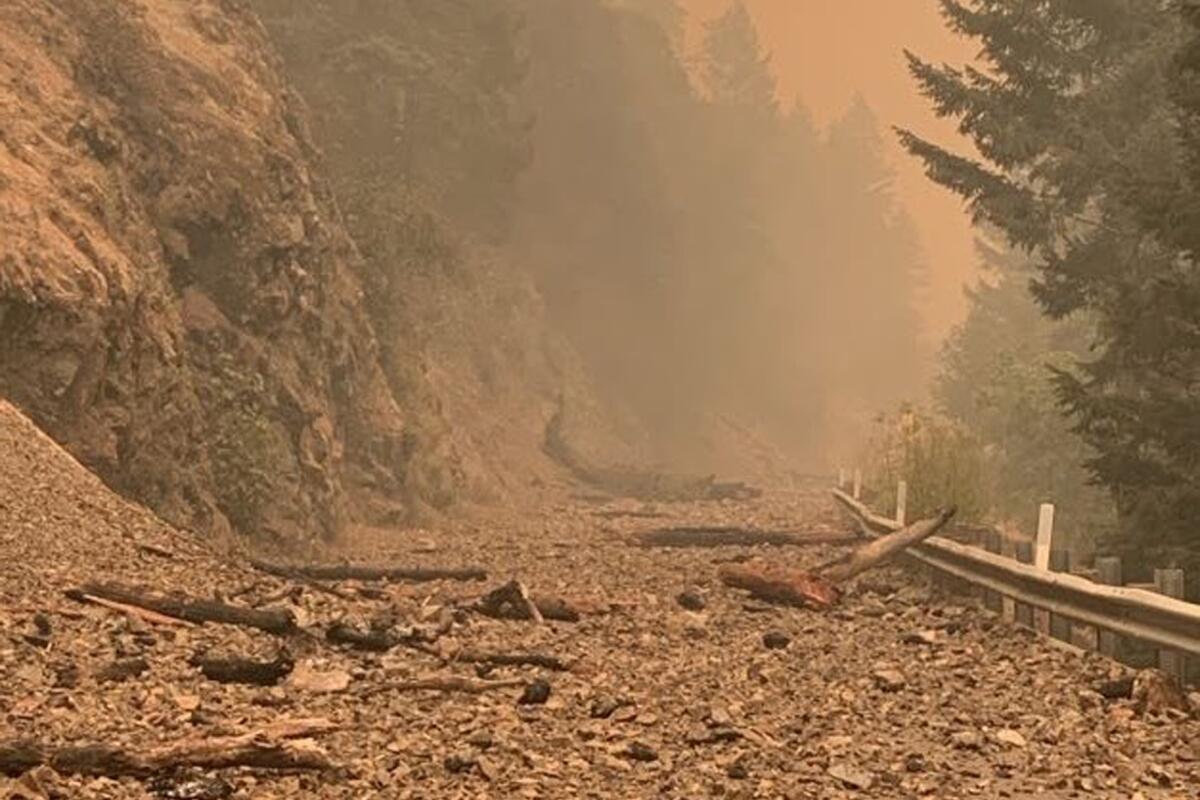The photograph appears to be an old, sepia-toned image that conveys a muted, reddish-brown color scheme, likely indicative of the period or due to a present smoke or haze, giving it a foggy appearance. The scene captures a rugged outdoor landscape during the daytime, characterized by a roadway that seems to have suffered the aftermath of an avalanche or possibly a wildfire. On the left side, the photograph shows a textured and rounded cliff of rocks with small stones appearing to slide down. The right side features a dense arrangement of trees with significant foliage, and in the far distance, more indistinct trees are visible through the thick fog. Additionally, a metal crash barrier, typical of those found on roads, runs along the right edge of the path, with a large branch resting against it. The ground is littered with numerous rocks, twigs, and broken, possibly burnt, tree branches, suggesting recent natural disruption. Overall, the image depicts a natural landscape disrupted by debris, with a contrasting man-made barrier and an atmosphere thick with haze and muted tones.